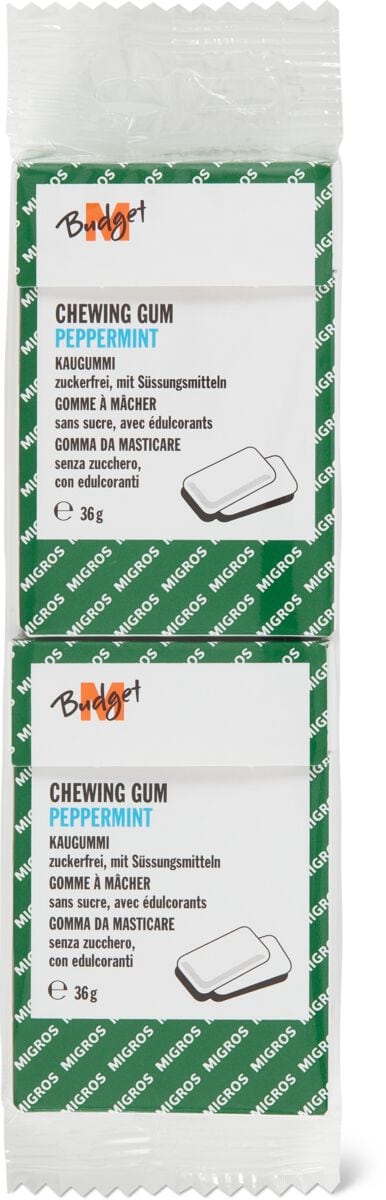The image shows two identical packages of chewing gum, joined in the middle by a plastic seam. Each package is made of plastic with plain white, jagged-edged sections at both the top and bottom. The main background of the packaging is green with the word "Migros" written repeatedly and diagonally in white text. At the top left of the label, there is an orange letter "N" followed by the word "Budget" in black letters, and beneath that, "Chewing Gum" in all capital letters. Further down, "Peppermint" is written in all capital turquoise letters. An illustration of two white rectangular gum pieces, resembling Chiclets, is present on each package. The label also includes the weight of the gum, indicated as "36 G." Additionally, there appears to be a list of ingredients, though they are not in English, making the specific contents unclear.